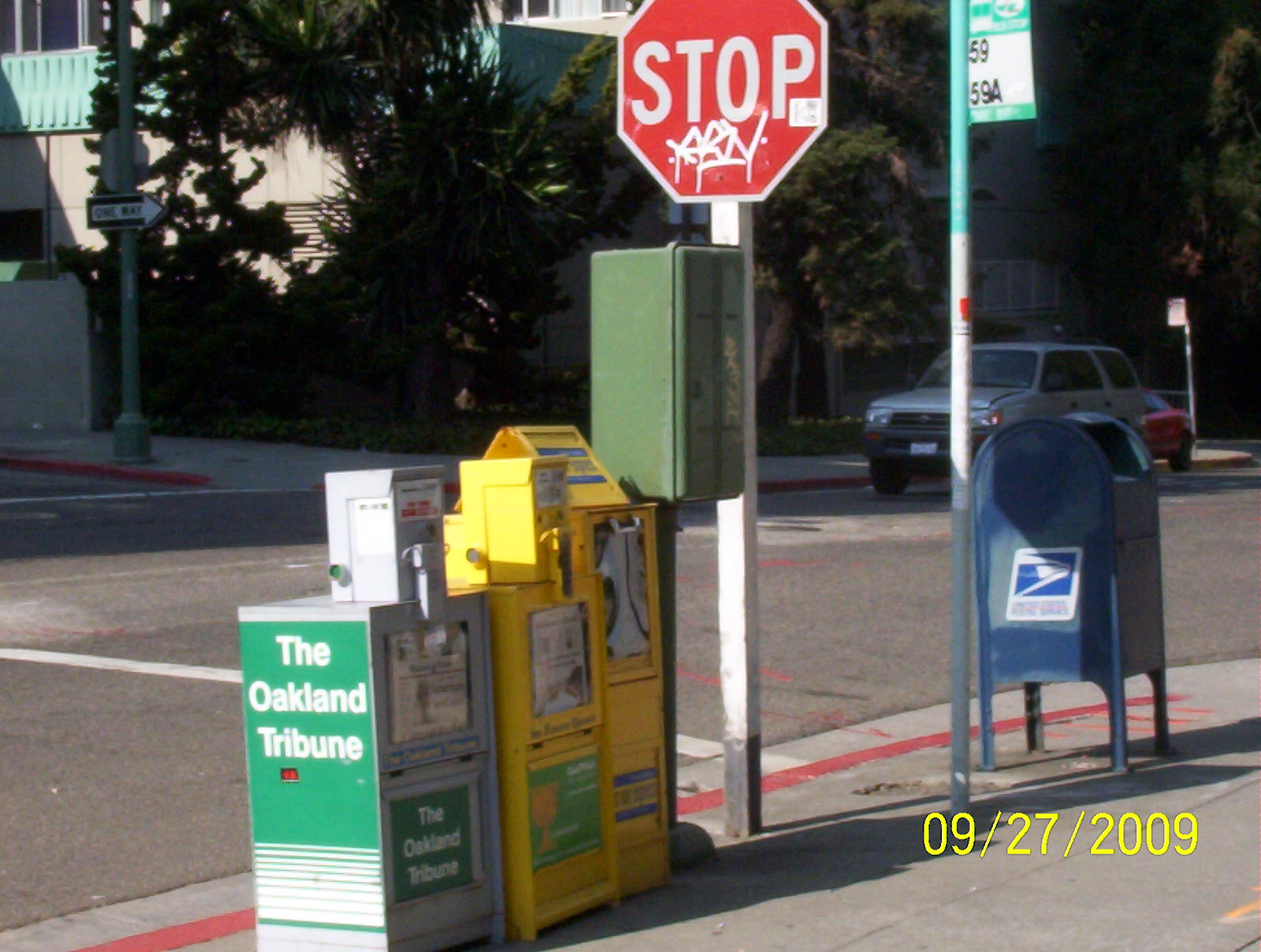The image captures a typical urban street scene dating back to September 27, 2009, as indicated by the date in yellow in the bottom right corner. Dominating the foreground on the left, there are several newspaper vending machines. The closest one is green with the white text "The Oakland Tribune," which also appears on the visible newspaper inside. Adjacent to this is a set of two yellow newspaper dispensers; one has a rectangular top and the other a square top. Flanking these vending machines is a tall, dark green plastic utility box with black lines on its front.

To the right of this setup, a stop sign, defaced with white graffiti, stands on a square pole. Slightly further along the street, there's a blue post office mailbox with the postal service logo and a rounded top. Behind the mailbox, a pole transitions from white at the bottom to light green at the top. The street itself is asphalt with a red line marking the curb and a white pedestrian crossing extending from the stop sign.

In the background, a light gray SUV with a white license plate is parked, and further back, the area is bordered by buildings with teal and concrete walls. A street sign on the far left points to the right, indicating a one-way direction. The overall scene is framed by hints of greenery and exudes the feel of a bustling urban environment in the late 2000s.